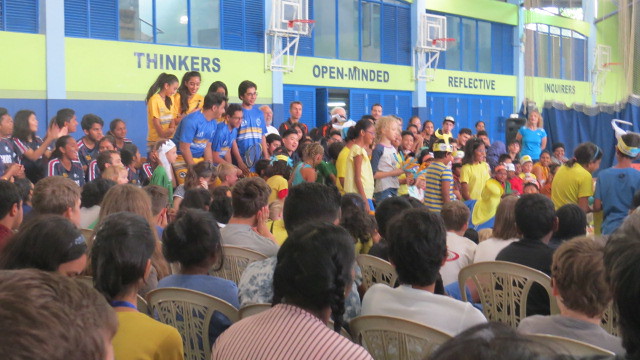This vibrant full-color photograph captures a lively school function with a bustling crowd of young students. At the center of the activity, a group of about two to three dozen students is both standing and seated on white chairs, creating a sense of community and engagement. While individual faces are indiscernible, the overall energy of the gathering is palpable. 

Dominating the background, signs hang prominently beside basketball hoops. These signs bear inspirational words like "Thinkers," "Open-minded," and "Reflective," with one sign partially obscured and unreadable. 

Toward the upper section of the image, a noticeable group of six children draws attention. This subgroup consists of three boys wearing blue outfits and three girls dressed in yellow, positioned slightly elevated above the rest of the crowd. This distinct placement suggests their involvement in a special award ceremony or program, adding an element of significance to their presence in the photograph.